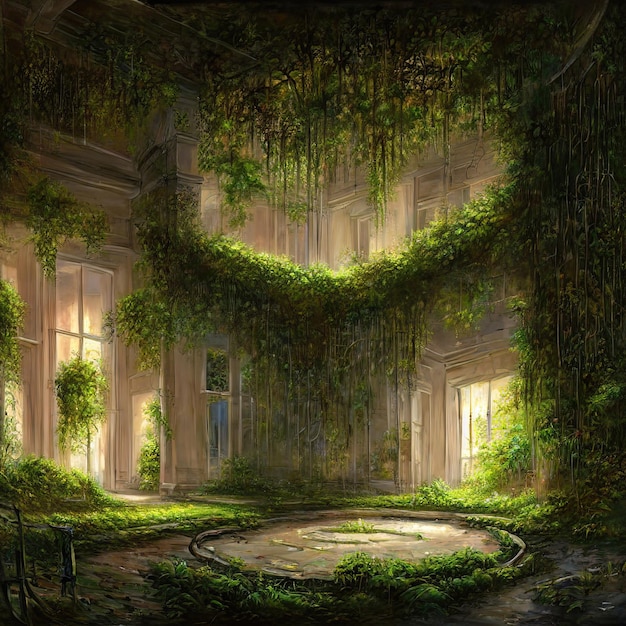This detailed painting depicts the interior of an aged, upscale building overtaken by nature, featuring tall ceilings and multiple windows streaming in daylight, creating a stark contrast against the predominantly dark and brown-colored walls and soil-covered floors. The room houses numerous plants, with grasses and foliage growing directly from the soil on the ground and encroaching on the building's walls. A prominent circular arrangement of stones lies in the center of the room, with plants sprouting along its circumference and in its middle. The left side shows tall windows with plants growing around and above them, alongside an open door revealing more greenery. Near these windows, plants hang from the ceiling. On the right, windows mirror this vegetation, and a stairway is flanked by trees. Both walls are adorned with green and brown vines trailing downwards. An opening in the ceiling reveals the floor above, from which more plants and vines dangle towards the ground floor.